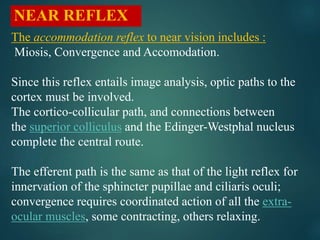The image is a square digital piece with a dark green background that gradually becomes lighter towards the center. It features left-aligned text. In the upper left corner, there is a red rectangular box with the words "NEAR REFLEX" written in bold, all-caps yellow letters. Beneath this, in gold writing, it says "The accommodation reflex to near vision includes" which is underlined. The remainder of the text is predominantly white, though a few terms are highlighted in green, specifically "superior colliculus" and "extraocular muscles."

The descriptive content reads: "Since this reflex entails image analysis, optic paths to the cortex must be involved. The corticocollicular path and connections between the superior colliculus and the Edinger-Westphal nucleus complete the central route. The efferent path is the same as that of the light reflex for innervation of the sphincter pupillae and ciliary muscles. Convergence requires coordinated action of all the extraocular muscles, with some contracting and others relaxing."

The overall style of the piece is digitally rendered, clearly designed to convey detailed information about the near reflex in a visually structured manner.